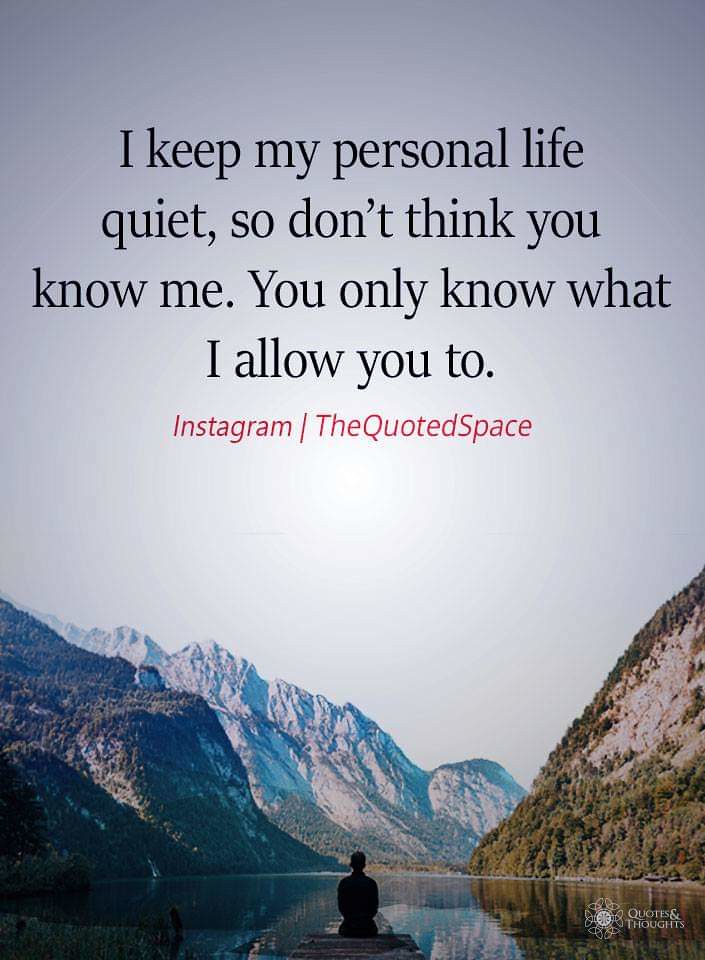The image is a vertical rectangular poster featuring an evocative natural scene overlaid with a poignant message. The bottom part of the image shows a serene body of water flowing through a mountain valley, with a silhouette of a person sitting on what could be a dock or a raft, their back turned to us, contemplating the tranquil nature. The mountains on either side of the river differ in texture; the left side appears more rocky while the right side is densely wooded. The reflections of these mountains are visible in the clear water. Above this scene, the sky shifts colors from a grayish blue to almost purple. In the upper part of the image, in bold black letters, is the quote, "I keep my personal life quiet so don't think you know me. You only know what I allow you to." Beneath the quote, in smaller red letters, it reads, "Instagram/theQuotedSpace."